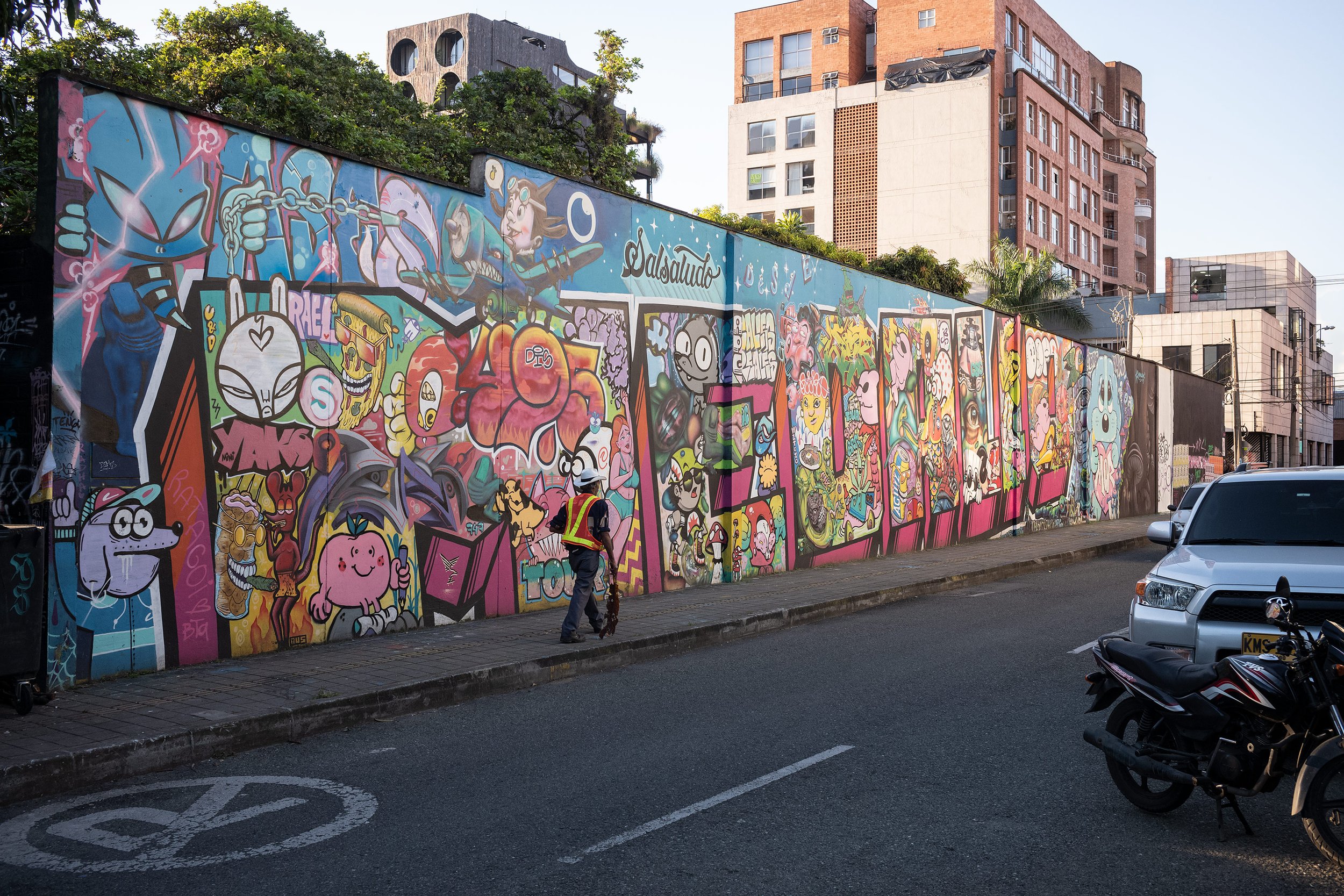This vivid city street captures a stunningly detailed mural stretching across a towering concrete wall, approximately 20 feet high and 60 to 100 feet long. The professionally done graffiti blends vibrant cartoony images with block letters that spell out "M-E-D-A-L-I-O." The background predominantly showcases shades of blue, enhancing the colorful array of characters within the mural. Notable details include a playful dog in the bottom left corner, adorned with a ball cap featuring a Nike emblem, light blue on its underside, long floppy ears, glasses, and a green and blue tracksuit. The mural also houses diverse and whimsical elements such as an alien, a face on an airplane, various animals, apples, and a yellow pizza. The scene is further animated by a man in an orange worker's vest walking along the sidewalk in front of the wall, heading towards the right, with tall buildings and trees rising in the backdrop, and a road visible in the bottom right portion of the image.